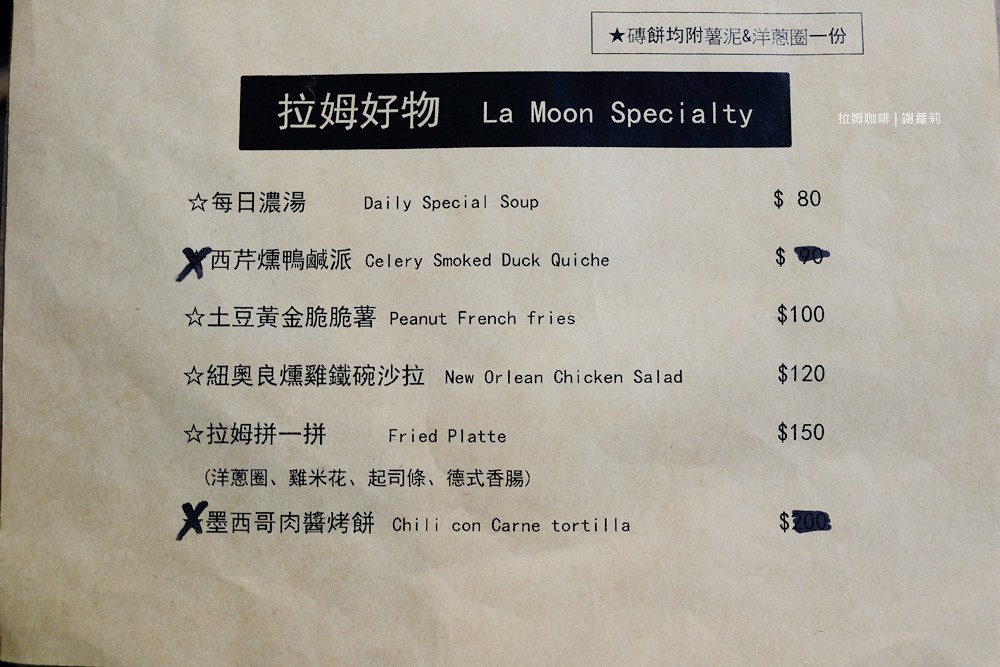The image is a detailed menu written predominantly in Mandarin Chinese characters, indicating it is likely from a Chinese restaurant. At the top of the image, there is a black box containing complex Chinese characters, alongside the text "Lamoon Specialty" in white. To the right of this box, there is additional white text in small Chinese characters.

Above this black box, there is another border box with a star symbol and more Chinese text. Below the black box, the menu is displayed in a structured manner. On the left side of the menu, rows of Chinese characters correspond to various menu items. There are six items listed, each row accompanied by a star symbol. Notably, the stars next to the second and last items are blacked out.

To the right of the Chinese characters, the menu lists the names and prices of the dishes in English:
1. **Daily Special Soup - $80**
2. **Celery Smoked Quiche - $90 (price blacked out)**
3. **Peanut French Fries - $100**
4. **New Orleans Chicken Salad - $120**
5. **Fried Plat - $150**
6. **Chili Con Carne Tortilla - $200 (price blacked out)**